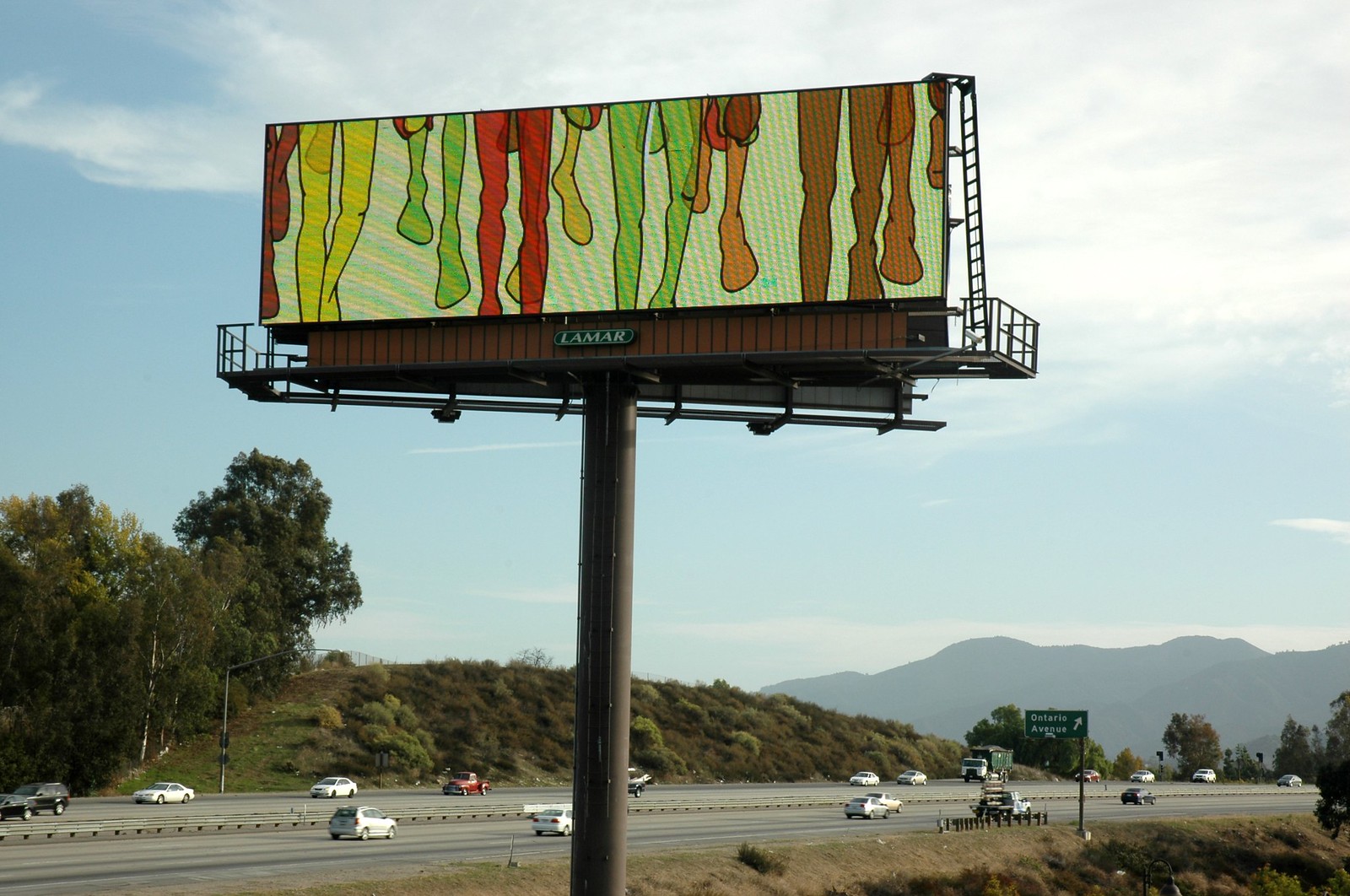In this rectangular daytime photograph, we observe a bustling interstate highway stretching from east to west. The highway features three to four lanes in each direction, separated by a sturdy guardrail. The road is teeming with cars traveling in both directions, highlighting the busy nature of this thoroughfare. In the background, a distant range of pale-colored mountains creates a serene backdrop, adding a sense of depth to the scene. Closer to the highway, a grassy area transitions to a cluster of trees on the left side, contributing a touch of greenery to the composition. Above, the sky is a light blue, interspersed with soft white clouds, adding to the overall serene yet dynamic atmosphere of the image.